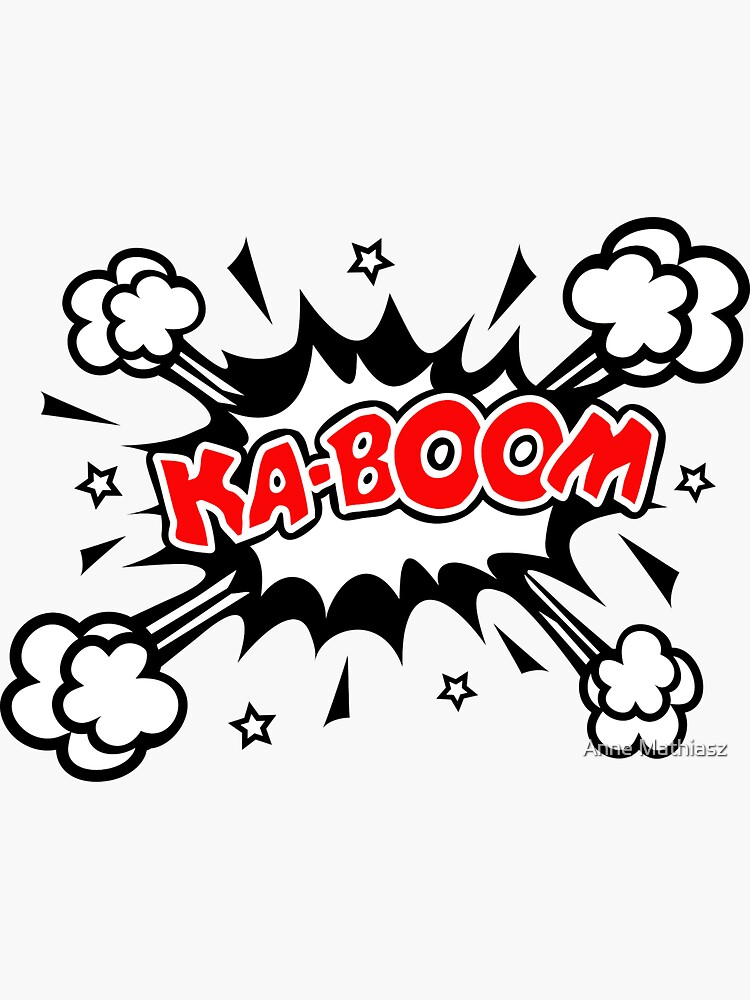This comic book-style illustration features a dramatic explosion set against a white background. The explosion is depicted with an oblong, jagged-edged burst in black, overlaid with a similar white burst, and surrounded by four puffs of smoke at each corner of the frame. In the center of the explosion, bold red letters spell out "KA-BOOM," outlined first in white and then in black. Small stars, white with black outlines, are scattered around the illustration, adding to the dynamic sense of impact. The word "Martinez" is inscribed in the bottom-right corner, completing the vibrant and energetic scene.